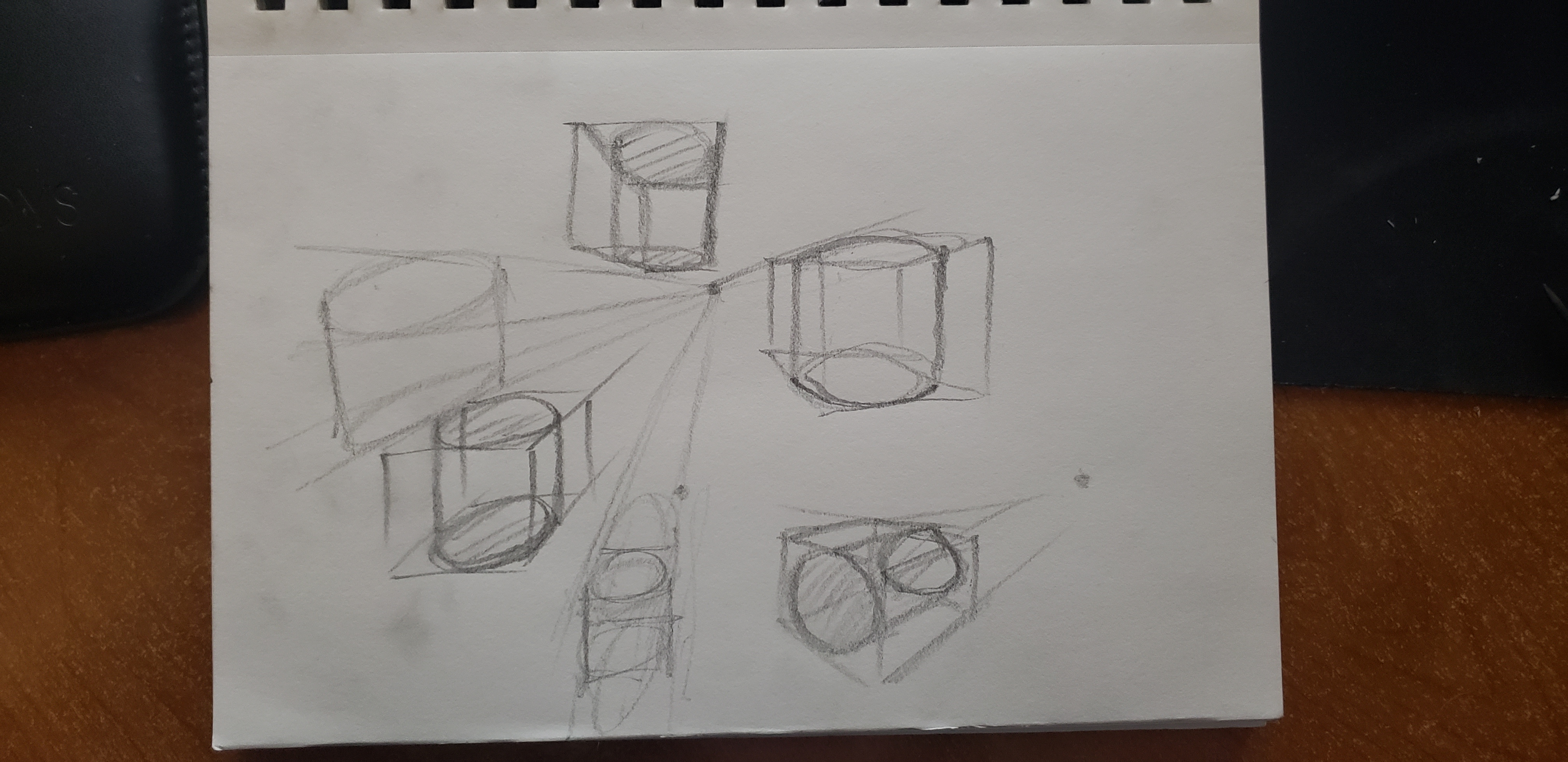This is an image of a white sketch pad that shows intricate pencil drawings of geometric shapes in various projections. The page features six distinct sketches of cylindrical objects, each depicted in a different perspective. The primary design element shows a small central circle with a short horizontal line angling slightly upwards to the right, connecting to another circle. Extending from this circle are two lines that lead downwards to a third circle enclosed within a square. This configuration is repeated in various orientations: one to the left above the center dot, three more aligned vertically on the left-hand side of the page, and one freestanding below and to the right of the other shapes. None of the shapes are filled in, though some lines are darker and feature shading to suggest depth. The sketch pad itself is propped on an orange-brown tabletop with a dark black background at the top of the image. Additionally, there are slightly cropped-out holes along the top of the paper, indicating that it could be from a notepad or folder. The detailed pencil work emphasizes the geometric form, showing the objects contained within cubes or box-like structures, including one with a conical, pyramidal shape.